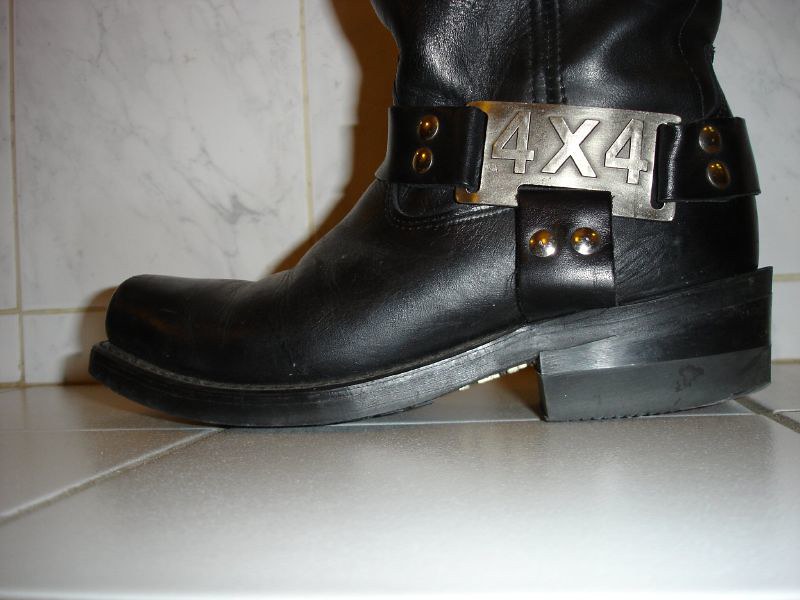This photograph showcases a close-up view of the bottom portion of a black leather motorcycle boot, positioned against a white tiled floor and a white marble-tiled wall. The boot features a small curved heel and several decorative leather straps wrapping around its ankle. Prominently, a rectangular silver metal piece, through which the leather straps are threaded, is emblazoned with the numbers "4x4". The photograph cuts off the upper part of the boot, leaving it partially visible.